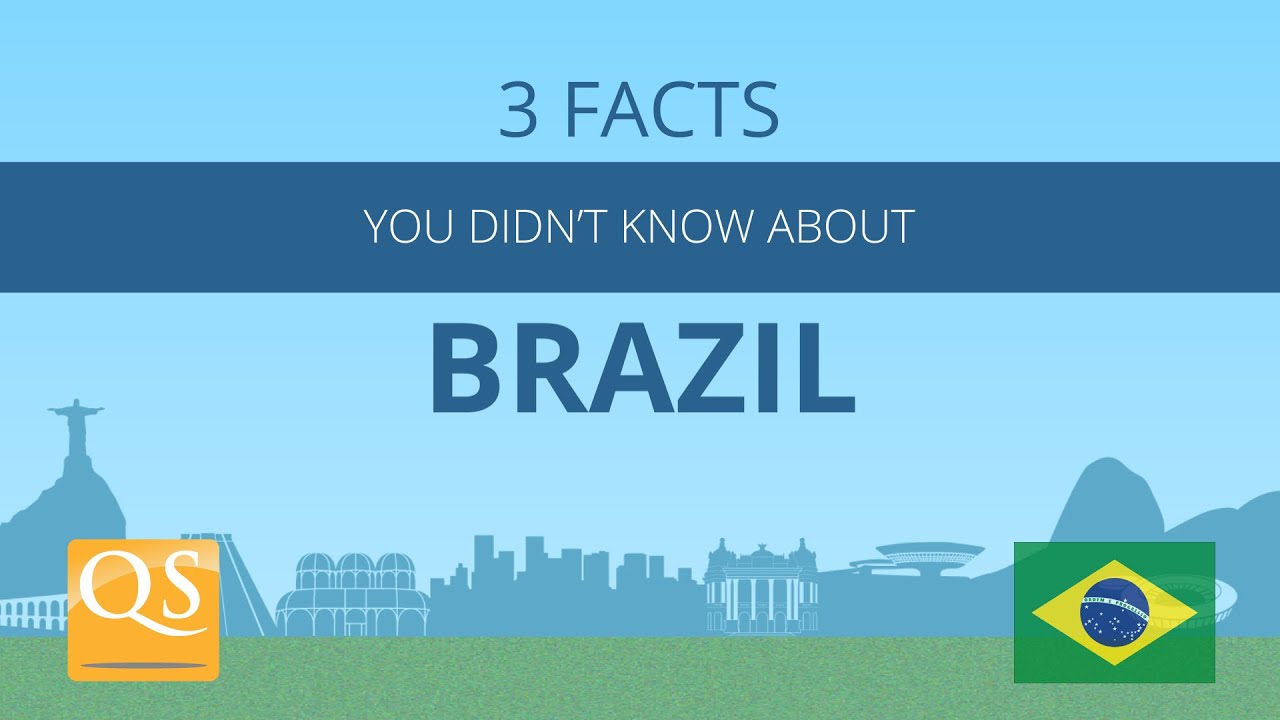The image appears to be an advertisement highlighting the attractions of Brazil. The background is a vibrant, bright light blue, almost teal color, creating a refreshing and inviting atmosphere. Within this background, multiple iconic images are displayed, including the towering statue of Christ the Redeemer with outstretched arms, various monuments, bustling restaurants, and scenic hills, all representative of Brazil's renowned landmarks and culture. Near the bottom portion, the background transitions to a slightly darker teal, with a strip of green below that resembling grass.

Prominently centered in the image, bold text in dark teal reads, "Three Facts You Didn't Know About Brazil," catching the eye. Additionally, the design incorporates a QS logo in an orange box on the left side, and a globe motif encased within a yellow diamond and a green square. The word "Brazil" and the phrase "Three Facts" are emphasized in dark teal, while "You Didn't Know About" is set against a teal rectangle spanning the width of the image, creating a cohesive and visually appealing layout.